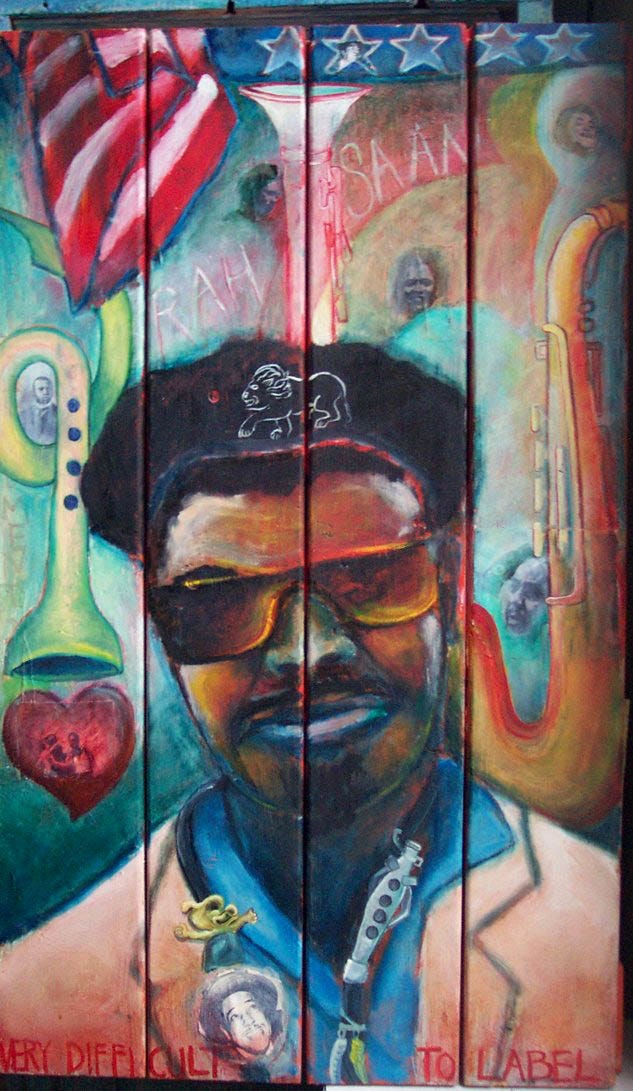The image is a color photograph in portrait orientation, depicting a detailed mural painted or drawn in chalk on a vertical wooden fence composed of four slats. The mural features an African-American man, possibly a figure connected to the Black Panther movement, occupying the bottom half of the image from the top of his head to mid-chest and from shoulder to shoulder. The man is wearing distinctive orange sunglasses and a peach-colored blazer over a blue collared shirt. He sports a black beret adorned with a white lion insignia and has various lapel buttons.

Surrounding the man are several vertical musical instruments: to his left, there is a downward-pointing green horn above a red heart, and to his right, an orange saxophone. Above the man's head, the name "Rah Saan" is inscribed in white chalk. In the top left corner of the mural is a partial view of a flag with red and white stripes and blue stars. At the bottom of the mural, in red letters, the phrase "Very Difficult to Label" is prominently displayed. The overall style of the mural combines elements of realism and representationalism, capturing the essence of outdoor chalk art.